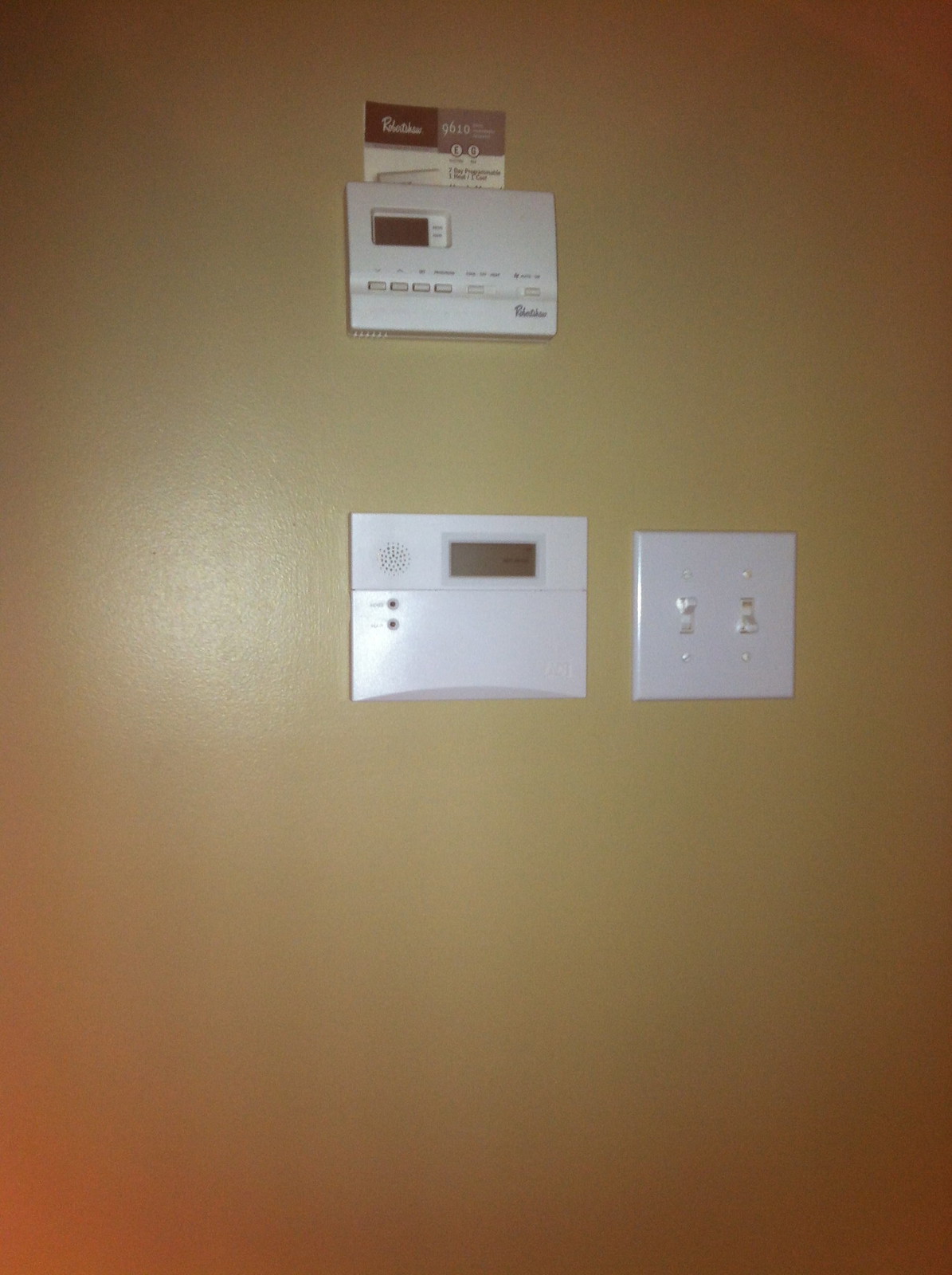‘A tan-colored wall adorned with three distinct objects: At the top, there's a white digital thermostat featuring a dark display panel that shows the temperature. The brand name is visible on the right side, though it's unreadable. The thermostat has four buttons below the display, and there appears to be a set of usage instructions tucked above it. Beneath the thermostat, there is another device which resembles a thermostat but could be an intercom due to its small speaker grill. It also has an unidentified display window with two tiny circles, likely indicator lights, beside it. Finally, to the right of these devices is a white light switch panel with two on/off switches. The overall color scheme includes shades of tan, white, black, and gray.’